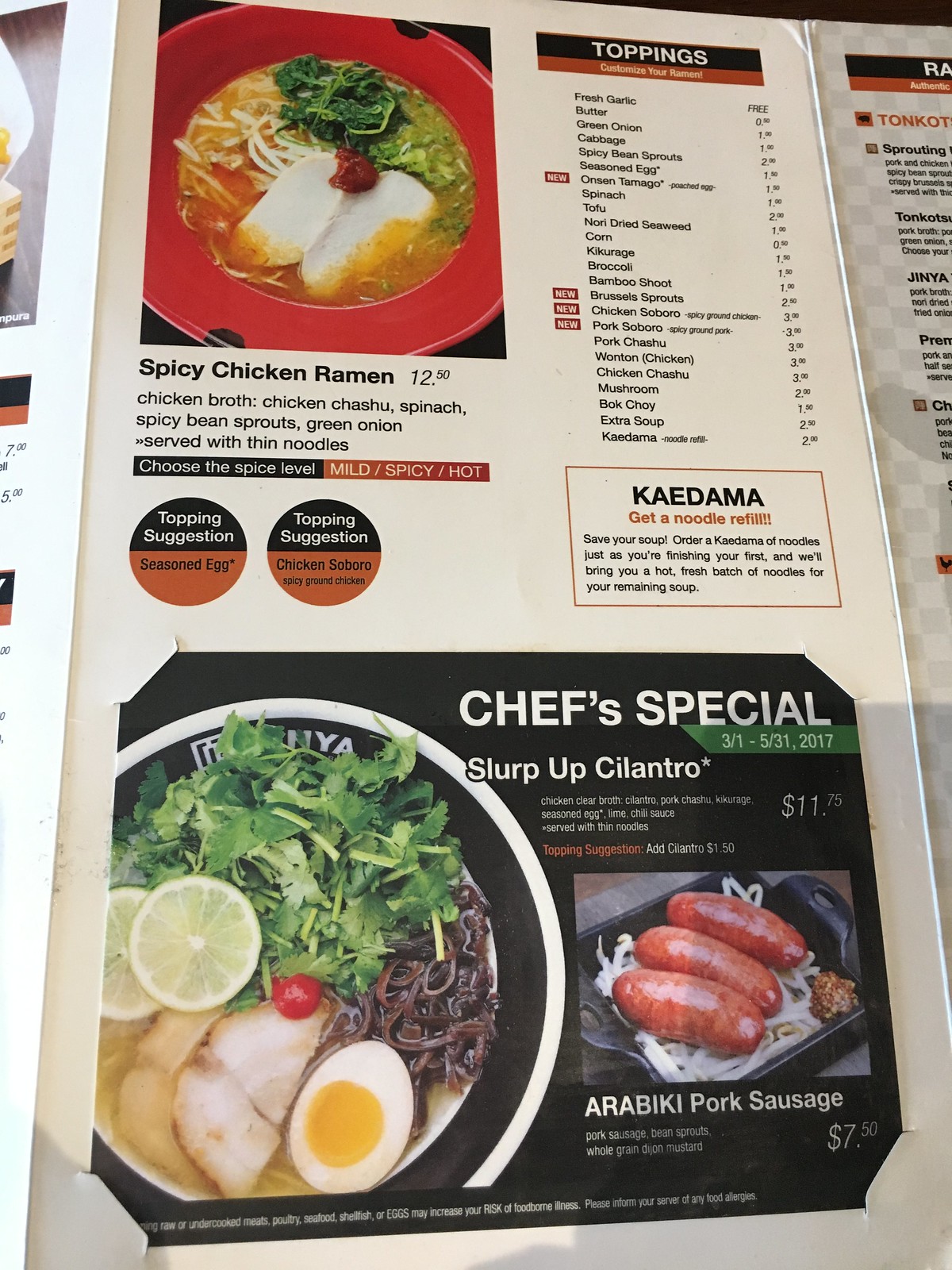The image features a detailed menu spread from a trifle restaurant, showcasing the middle pages. The left and right sides of the menu are visible, though the menu on the right side is partly cut off and displayed against a gray and white checkered background. On the left side, there is a white section with an image whose details are indistinguishable.

At the top left of the menu, an enticing image highlights the "Spicy Chicken Ramen," priced at $12.50. This dish includes a flavorful combination of chicken broth, chicken chashu, spinach, spicy bean sprouts, green onion, and thin noodles. Customers can customize the spice level to be mild, spicy, or hot. Recommended toppings include seasoned egg and chicken chashu.

On the top right, the menu lists a variety of toppings for ramen customization, including fresh garlic, butter, green onion, cabbage, spicy bean sprout, seasoned egg, naruto (fish cake), tofu, dried seaweed, corn, cucumbers, broccoli, bamboo shoots, brussels sprouts, and more. Additionally, various protein options like chicken chashu, pork chashu, pork shabu, fried wonton, chicken, mushroom, bok choy, and extra soup can be added. The option for a noodle refill, termed "Kaedama," allows patrons to enjoy a fresh batch of noodles with their remaining soup.

Below these sections, a large image showcases the "Chef's Special" - "Slurp Up Cilantro," priced at $11.75. Adjacent to this, another dish titled "Arabica Pork Sausage," priced at $7.50, features three plump sausages served on a bed of noodles in a sleek black square dish.

On the left side of the image, the "Chef's Special" appears to include chopped greens, black noodles, half an egg, what seems to be fish or chicken, a couple of lime slices, and a cherry tomato. This visually arresting presentation enhances the appeal of the menu, enticing diners with its vibrant and detailed culinary offerings.